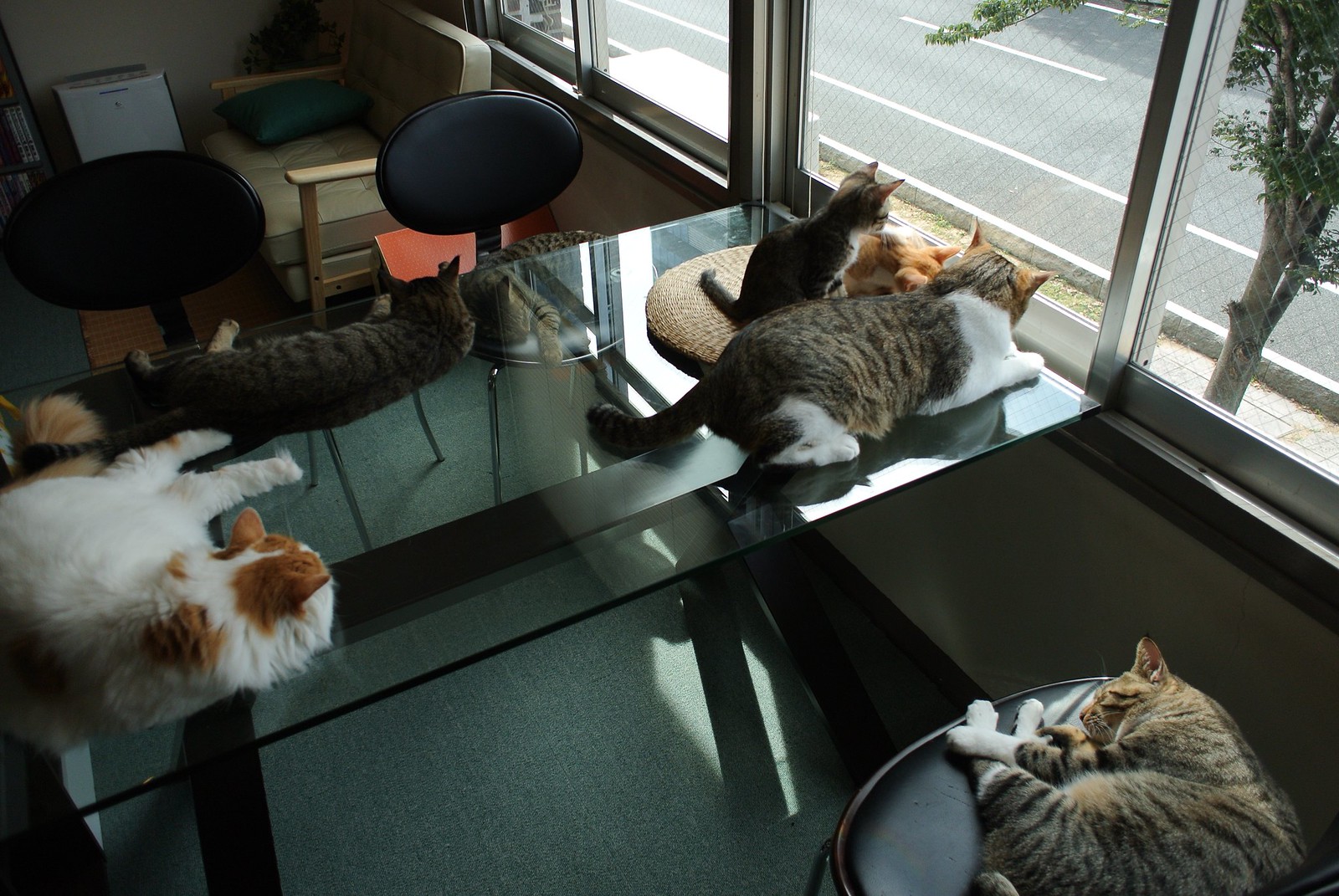This image depicts a sunlit office space, likely on the second or third floor of a building. Prominent in the scene is a sleek glass desk extending from a silver-framed, aluminum slider window with four panels, down to the left side of the room. The backdrop features beige-colored walls and gray carpet flooring.

Positioned around the glass table are various seating arrangements, including two black faux leather office chairs with round backs and steel legs, offering a contrast with a longer, beige armchair visible towards the back of the room.

Adorning the glass table and chairs, a multitude of cats can be seen. A notable cluster of four cats is resting atop the table. Two of these cats, one with a white body and orange markings, and another gray feline, are attentively gazing out of the window. Another cat, with brown and white fur, displaying a mostly white underbelly and brown ears, lies serenely on its side. By the table's edge, yet another cat, brown with grayish stripes and white paws, is comfortably settled on a circular object beneath the table.

Adding to the feline presence, a pair of tiger-striped cats lounge opposite each other on the chairs, their markings evoking the patterns of a wild leopard. An orange and gray kitten also joins the scene, peeking curiously out of the window from the table's surface.

This detailed tableau captures the coexistence of a professional office environment with the whimsical presence of these lounging and playful cats.